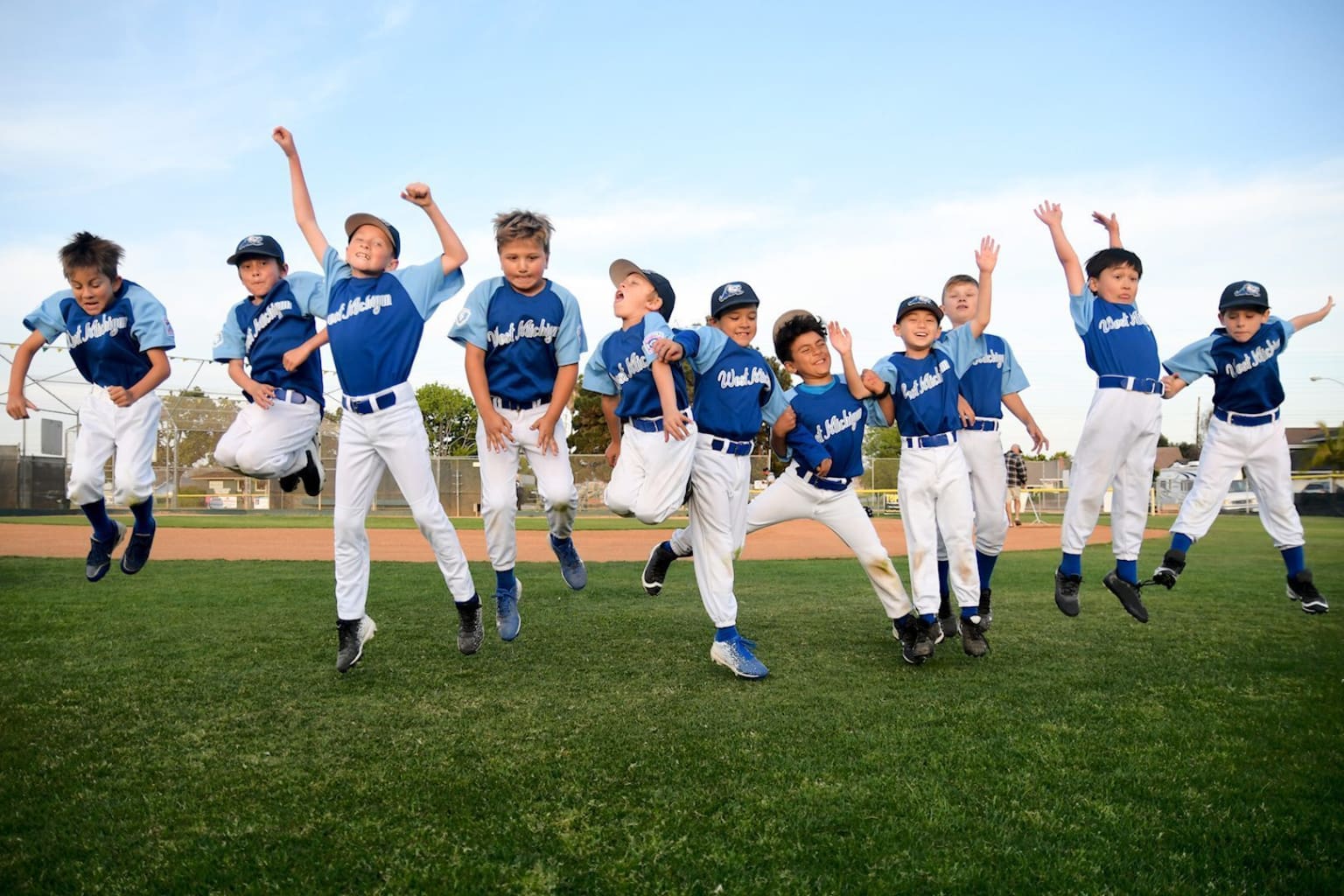In this vibrant photograph, a jubilant young boys' baseball team celebrates by enthusiastically jumping in the air for a team photo. Each player is dressed in a striking uniform featuring dark blue jerseys with light blue sleeves and white lettering, complemented by white pants secured with black belts. While most players sport black shoes paired with blue socks, a few stand out with blue shoes. Their outfits, though mostly clean, show signs of a well-fought game with a couple of players displaying dirt and grass stains.

The team stands on a well-manicured grassy section of a baseball field, with the dirt infield and bases visible behind them. Further back, a protective fence marks the boundary of the field, beyond which tall trees stretch up towards the sky. The backdrop is a serene blue sky adorned with wispy white clouds, adding to the cheerful atmosphere of the scene. Baseball caps in dark hues add a finishing touch to their uniforms, giving the image a cohesive look. This snapshot captures the essence of youthful excitement and team spirit on a clear, sunny day at the ballpark.